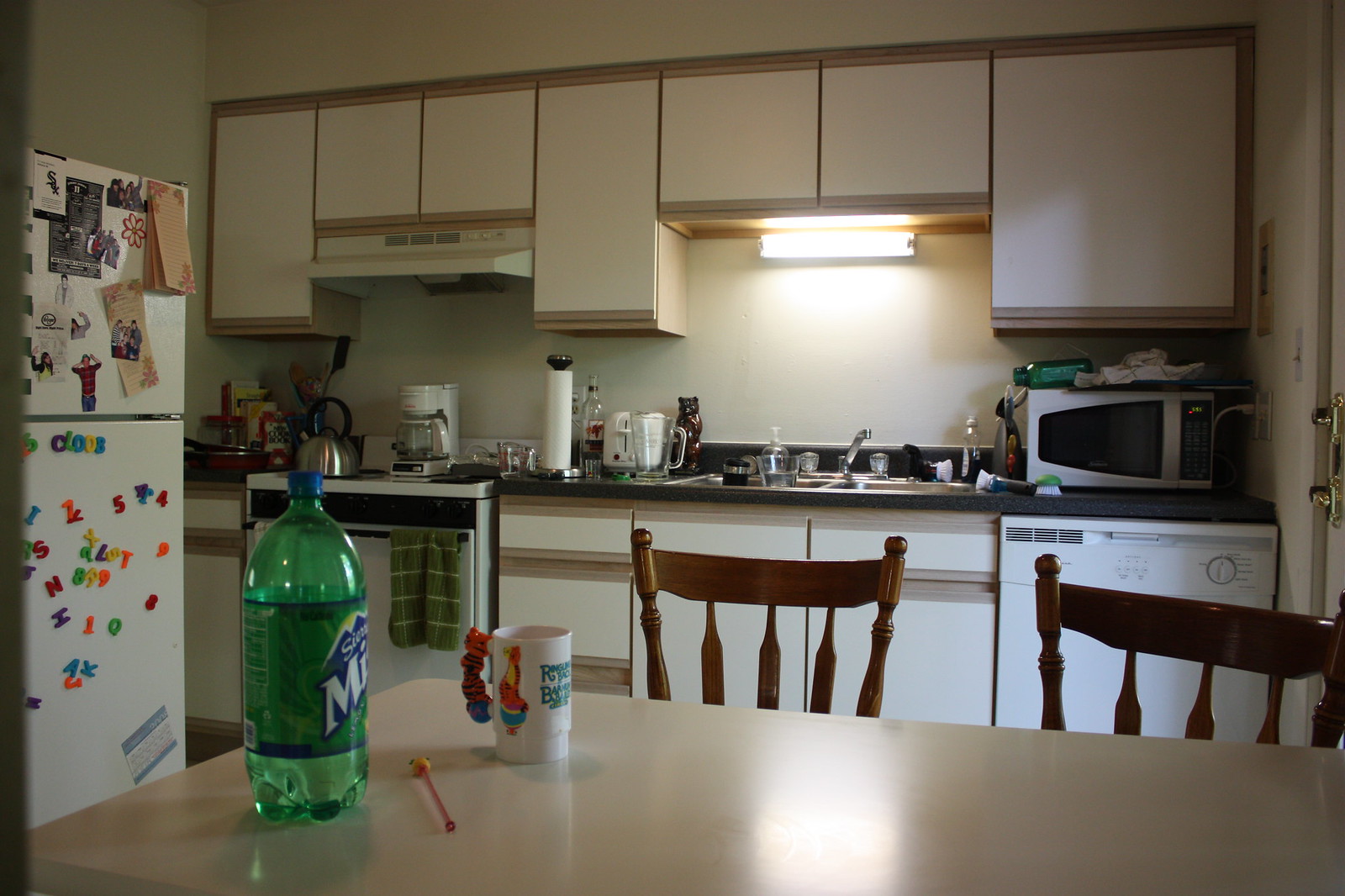This photograph depicts a cozy, compact kitchen that is meticulously neat and tidy. All the cupboards are positioned along one wall in the background, featuring a cream color with light brown trim and no hardware for a sleek look; these open by reaching the edge of the door itself. Above the white electric stove with black burners, there's a two-switch vent fan. This is a non-external venting type with louvers that recirculate air back into the room. One switch controls the two-speed fan, while the other operates the light fixture within the vent fan.

To the far right of the cupboards, a dishwasher seamlessly integrates into the layout. The dark countertop is adorned with a slight pebble pattern, exuding a subtle gritty look reminiscent of the late 1980s or 1990s aesthetic. A double stainless steel sink sits below a fluorescent light fixture tucked in the cove above it, providing ample illumination.

An off-white background ambiance complements the cream-colored cupboards. To the left of the image, a white refrigerator stands adorned with numerous magnets and items taped to its surface, showcasing a touch of personal flair. At the base of the image, there's what appears to be a breakfast bar that functions as a kitchen table. The synthetic surface holds an ornamental beaker, a mug, a straw featuring a cartoon character, and a bottle of Sierra Mist.

Multiple kitchen appliances are strategically placed on the countertop, including blenders, paper towel dispensers, coffee makers, a pot for boiling water, and a white microwave nestled in the right corner of the kitchen cupboard. This well-organized space exudes warmth and functionality within its compact design.